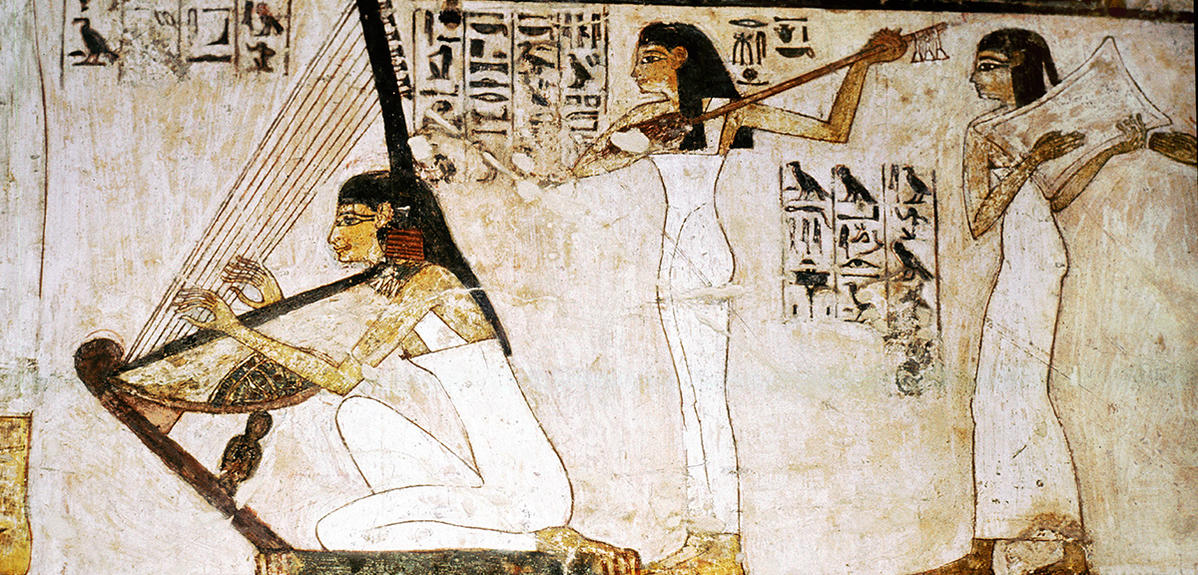This detailed illustration, likely painted on papyrus or an excavated ancient Egyptian wall, showcases three Egyptian women depicted in lively color, though the paint is flaked and slightly dirty from age. The mural, adorned with hieroglyphics in three distinct spots, portrays the women in the traditional Egyptian style with long, black hair and exaggerated eye makeup. Each woman dons a long, narrow white dress with thin straps.

Starting from the left, the first woman is kneeling and playing an ancient harp-like instrument, her hands extended delicately over the strings. The middle woman stands with a slightly damaged sphere that has bells hanging from one end, obscuring its full form. The woman on the right holds a vaguely square or rectangular object, reminiscent of a pillow, close to her face as she stands tall in profile, facing left. The muted white background with orange accents adds to the timeless authenticity of this ancient scene, capturing a moment from a distant past vividly and intricately.